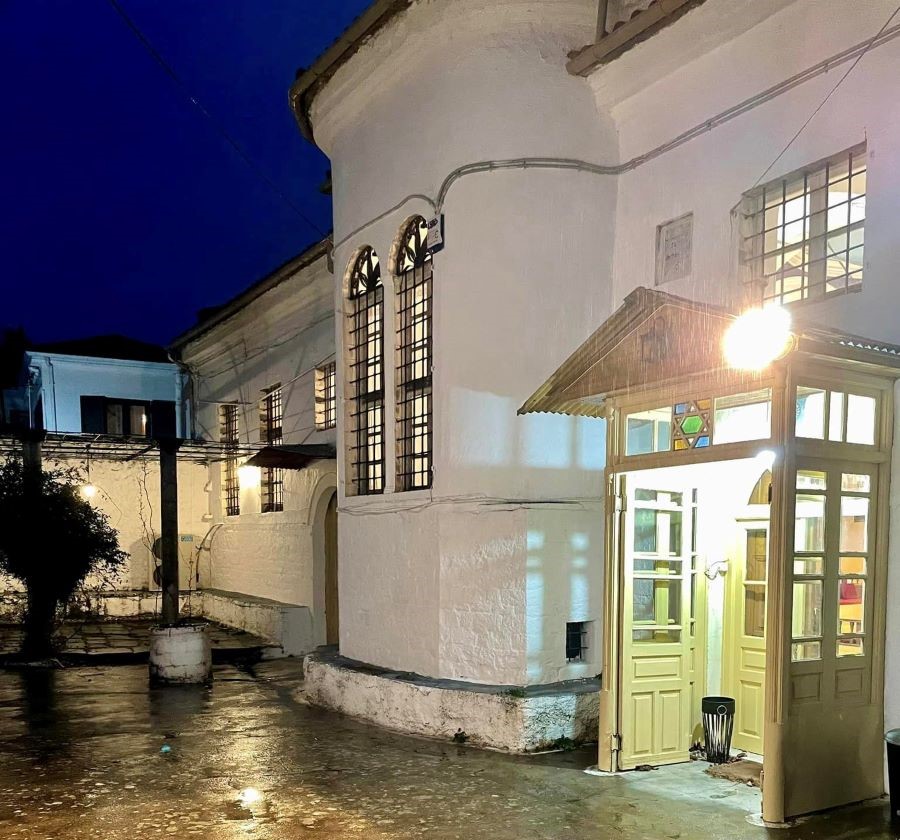This nighttime photograph captures a serene urban scene featuring a white-painted brick building with character-defining elements. Situated slightly to the right, the building exhibits a series of ornate windows adorned with black metal bars and dividers, lending it a checkered appearance. Protruding outward, some of these windows are elegantly arched, enhancing the building's architectural charm.

Dominating the entrance is a set of double wooden doors, the first of which is open, exuding a welcoming aura. Above these doors is a structure featuring the Star of David, hinting that the building might serve as a temple or place of worship. A covering extends above the doorway, designed to shield visitors from the rain.

To the right, a large streetlamp casts a luminous glow, illuminating the wet, reflective gray pavement below, suggesting a recent rainfall. The street's shininess under the warm light of the streetlamp captures a tranquil, freshly-rained-on atmosphere. On the left, a dark shrub or bush subtly frames the scene, along with a curious white bucket-like structure in the background, adding to the overall nocturnal ambiance.